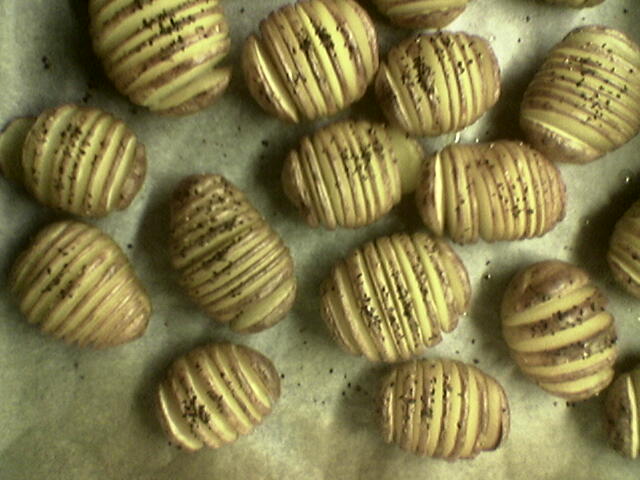The image displays a tray of at least 17 unpeeled potatoes that have been spiral cut but not yet separated into individual spiral pieces. The seasoned cuts, lightly dusted with what appears to be salt and pepper, clearly stand out along the circular slices. The silver tray holding the potatoes suggests that the dish could be prepared for a large family gathering or a meal at a restaurant. The retained skins on the potatoes give them a rustic appearance, indicating they were not peeled before the spiral cutting process.